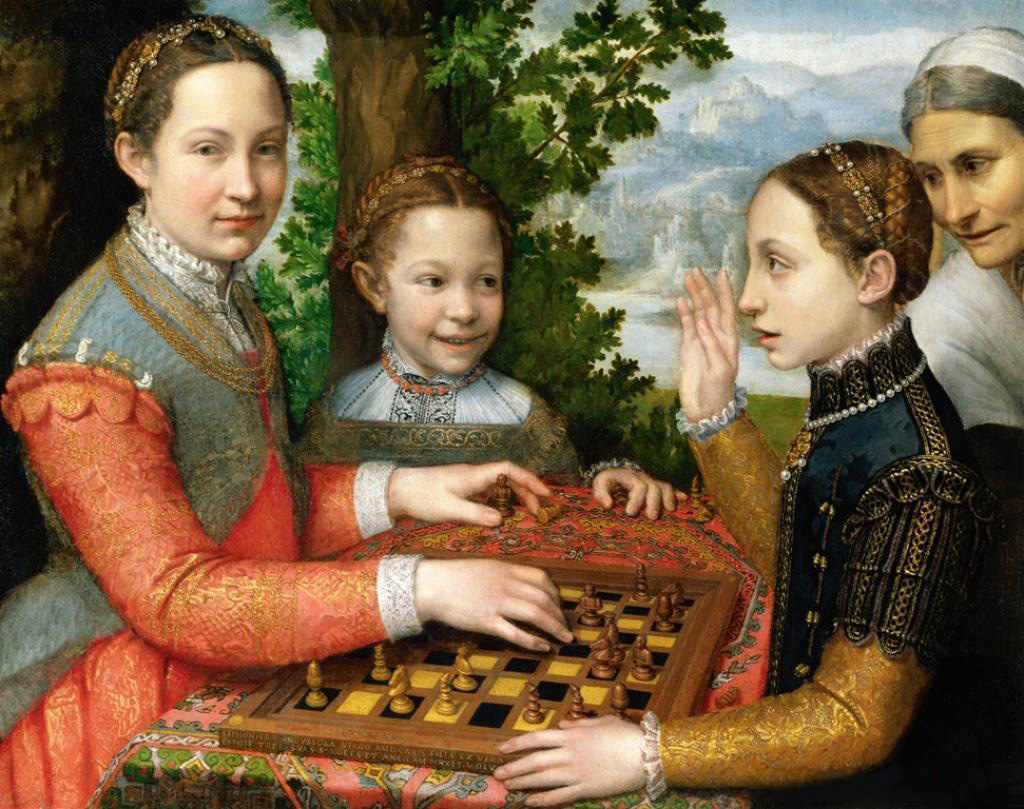In this detailed medieval painting, four women of varying ages are depicted around an ornately decorated chess set placed outside against a scenic background of trees, a river, and distant mountains. On the left, a dignified woman dressed in a luxurious bluish-orange gown with a tiara and necklaces sits at the table, her braid woven into a crown atop her head, and gazes directly at the viewer. Opposite her, another young woman in similarly regal attire concentrates on the chessboard, her right arm raised for reasons unknown. Between them, a cheerful young girl with a high-collar dress and braided hair stands off to the side, stealing the scene with her mischievous smile directed at the older sister-like figure. To the far right, an older woman, perhaps a servant, watches the game intently. The sunny outdoor setting with lush greenery and calming waters enhances the medieval aura of this engaging tableau.